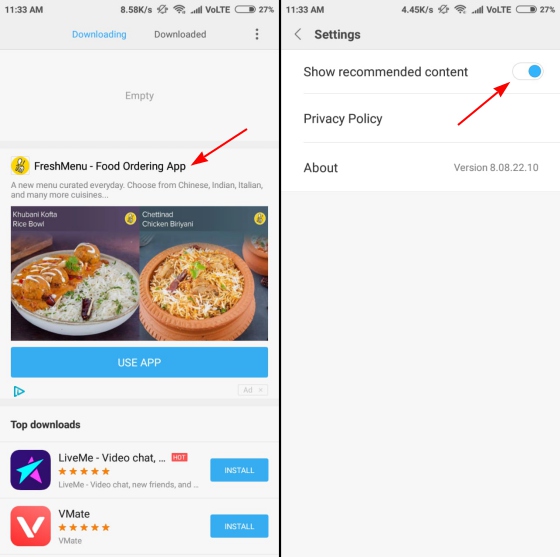This image captures two phone screens side by side. On the left screen, the top status bar displays the time, 11:33 AM, along with various symbols in a small font. Notably, the battery symbol indicates 27% battery life with a mostly white icon and a small black bar. Next to it, the words "downloading" in blue and "downloaded" in gray are visible, followed by three vertical dots. Below this status bar, there is a prominent white space with the word "empty" written in light gray text.

Under this white space, there's a yellow circle symbol with indistinct white and black details inside it, labeled "Fresh Menu - Food Ordering App." A red arrow points to this section. Below the label, a description reads, "A new menu curated every day. Choose from Chinese, Indian, Italian, and many more cuisines." Accompanying this text are two images of food plated against colored backgrounds—one with a purple backdrop and one with a blue backdrop. Beneath these images is a blue bar featuring the text "Use App" in white lettering.

At the bottom, the words "Top Downloads" are highlighted in bold black text, followed by a list of two apps. 

All these elements together create a comprehensive snapshot of a bustling phone screen promoting a food ordering app while displaying essential device information.